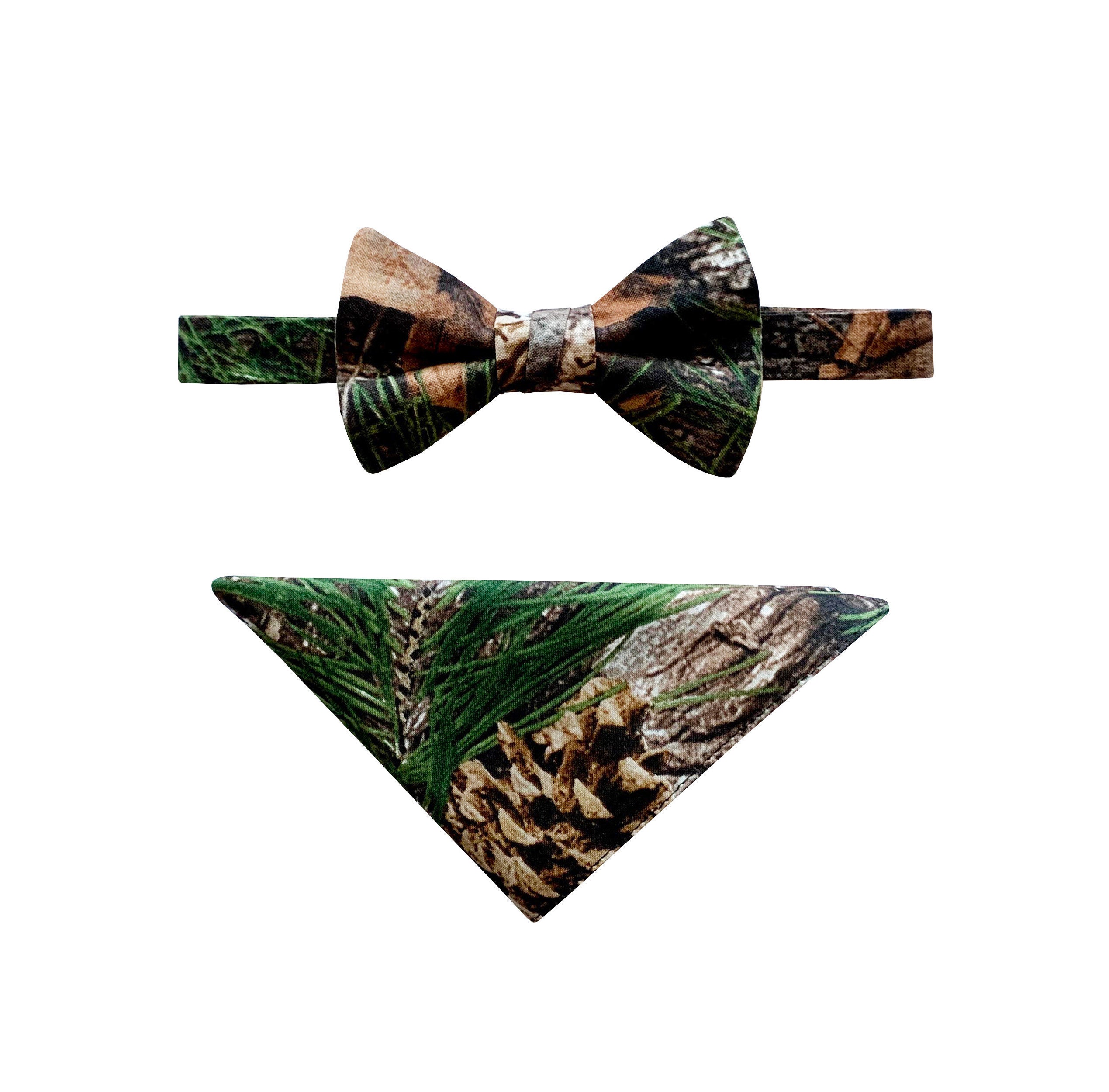The image showcases two matching clothing accessories featuring a detailed pine tree motif. The top accessory is a bow tie adorned with a comprehensive print of a pine branch, a large pine cone, and part of a tree trunk, although the design is not entirely visible due to the way the bow tie is tied. Below it, there's a triangular piece of cloth, presumably a handkerchief or pocket square, which prominently displays the same intricate pine tree design. Both items appear to be real, not digital renderings, and are set against a plain white background, suggesting they could be part of an advertisement for a clothing shop specializing in nature-inspired designs. The pine tree pattern wraps around the sides of both items, adding a cohesive and realistic touch to the overall outdoor aesthetic.